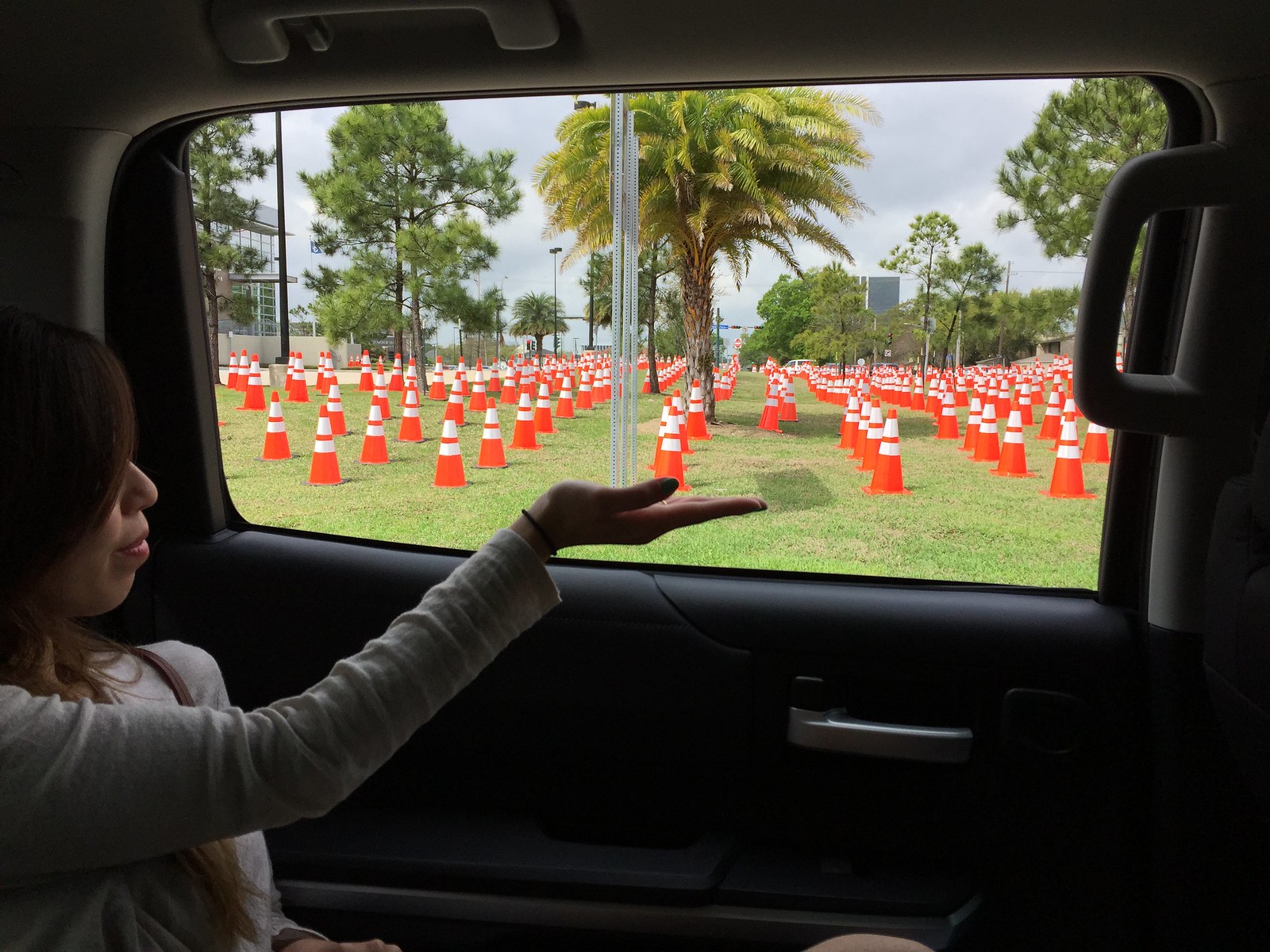Inside a car, a young girl with brownish, slightly reddish hair is captured in a side profile view, wearing a white shirt, holding her right arm up close to the window. The interior of the vehicle is black and gray. She seems to be humorously gesturing as if she is holding a small orange construction cone in her palm, her hand positioned an inch or two above where the window starts. Outside the car, there are multiple rows of orange traffic cones, each adorned with two white rings near the top, spread across a lush, grassy area. Surrounding the field is a variety of trees, including both palm-like trees and pine trees, contributing to a scenic backdrop. In the distance, there are glimpses of buildings nestled among the trees, with the ocean visible beyond them. The overcast sky casts a gray hue over the scene, enhancing the contrast of the vibrant orange cones. Street lamps are also visible, dotting the background. The girl's slight smile suggests a playful moment amidst the structured outdoor setting.